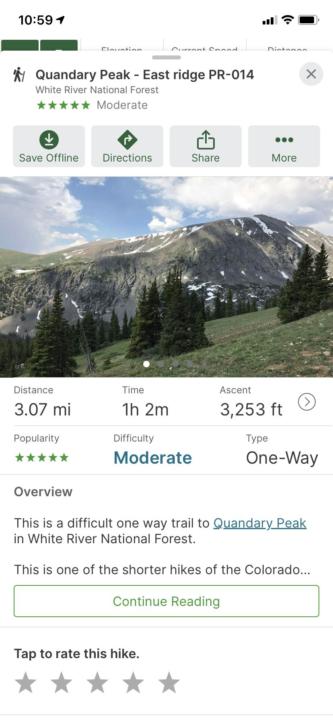**Image Description: Quandary Peak Trail Information**

The image captures extensive details about the Quandary Peak, East Ridge trail, and related statistics. The interface showcases a comprehensive informational layout:

- **Location Services**: Enabled, showing a reading of 1059.
- **User Ratings**: The trail has received 384 stars.
- **Connectivity and Battery**: Full Wi-Fi symbol indicating strong connectivity and an almost full battery icon.
- **Trail Name and Overview**:
  - **Quandary Peak, East Ridge**: Highlighted in green.
  - **Public Ratings**: 14 individuals have rated the trail.
  - **Area**: Located within the White River National Forest.
- **User Interaction Options**:
  - **Ratings**: An average rating of five stars is visible.
  - **Offline Availability**: Users can save the trail information for offline use.
  - **Directions**: Access to navigation directions.
  - **Additional Information**: A button for accessing more details.
- **Trail Visuals**: A captivating image of the trail featuring a mountain against a backdrop of blue sky, scattered white clouds, surrounded by trees, and a dirt pathway.
  
**Trail Statistics**:
- **Distance**: 3.07 miles.
- **Estimated Duration**: 1 hour and 2 minutes.
- **Elevation Gain**: 3,253 feet.
- **Trail Popularity**: Rated with five stars.

**Trail Difficulty**: Moderate.
**Type**: One-way trail.
**Overview**: This route is described as a challenging one-way trail leading to the summit of Quandary Peak within the White River National Forest. It's noted as one of the shorter hiking options in Colorado.

**Engagement Prompts**:
- **Continue Reading**: An option to read further details.
- **Rating Call-to-Action**: Users can rate the trail by tapping to provide a rating from 1 to 5 stars, with a current average of great reviews.

The detailed caption provides an extensive and informative view of the trail, appealing to avid hikers and nature enthusiasts looking for their next adventure.